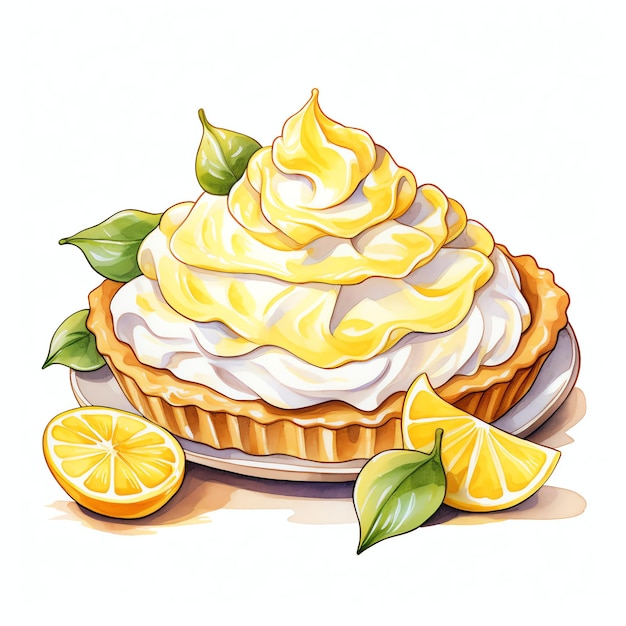This image is a detailed drawing, possibly a watercolor, of a lemon meringue pie. The whole pie, with its flaky light brown crust, rests on a white platter at the center of the composition. Topping the pie is a high, fluffy, toasted meringue that has a slight yellow-browned effect from being baked. In front of the pie are two yellow lemons; one lemon is halved and sits cut side up to the left, while the other is a quarter section positioned on the right. Scattered around are multiple green leaves—one near the halved lemon, another adjacent to the quarter slice, and three more behind the pie. These leaves add a touch of greenery and could be either lemon or mint leaves. The drawing is purely illustrative with no text or people depicted.